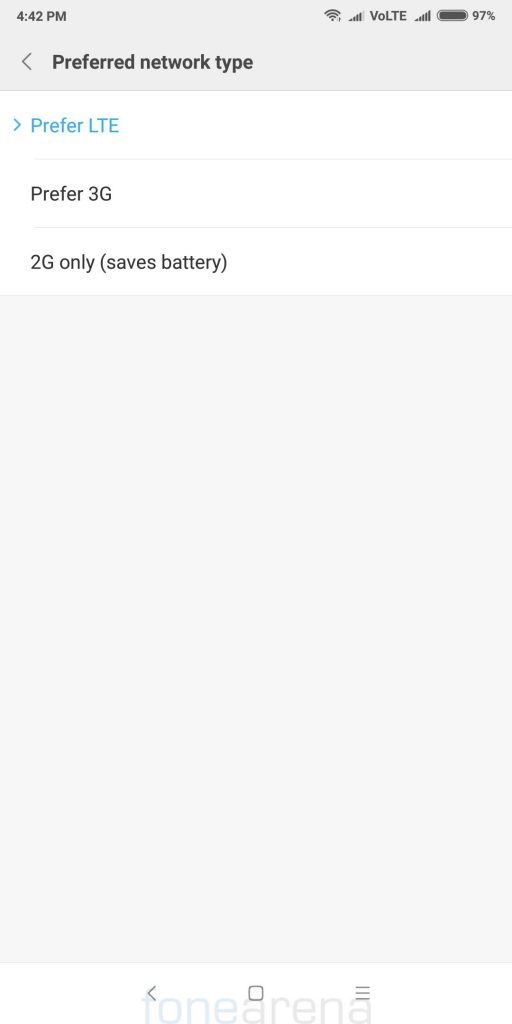The image is a screenshot from a mobile device. The status bar at the top indicates the time as 4:42 PM, with the icons showing full signal strength for both cellular and Wi-Fi connections, and a battery level at 90%. The screen is displaying a settings page for network preferences. There are options listed in a column: "Preferred network type" with choices such as "LTE preferred," "3G," and "2G only (saves battery)". The "LTE preferred" option is selected, highlighted in blue. 

The background of the screen features varying shades of white and gray. The upper section, where "Preferred network type" is located, is a lighter gray, transitioning to a pure white beneath the options list. The lower part of the interface contains navigation buttons: a left-facing arrow, a square, and an icon with three stacked horizontal lines. At the bottom of the screen, the text "PhoneArena" is displayed in a very light, almost indistinct gray or brown color against the off-white background. The predominant colors on the screen are blue, black, white, gray, and possibly a faint brown.